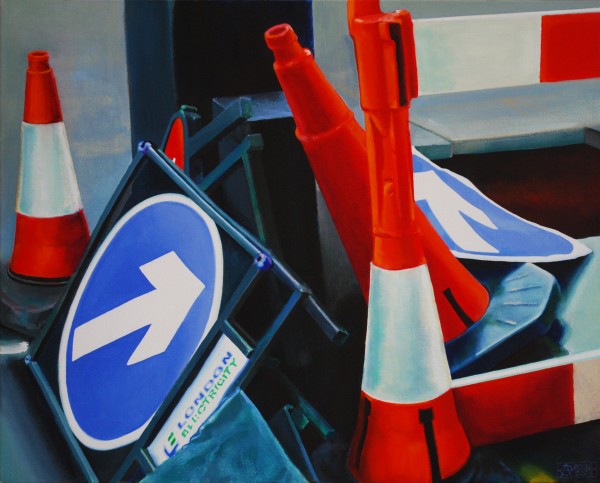The image captures a somewhat close-up view of a section that resembles a parking area. To the left, there is a prominent orange traffic cone with white and orange stripes on a black square base. In front of it stands another cone, entirely orange, and behind it, several other similar cones are visible. Additionally, there's an orange and white barrier or striped item that appears to demarcate a specific area. 

Nearby, a small metallic sign with a white circular border features a large white arrow pointing diagonally to the right on a blue background. This sign is lying down, possibly toppled over. To the right of this setup, a gray ledge is visible. Overall, the scene is characterized by various cones and signs, suggesting a regulated space, potentially a parking lot or similar area.